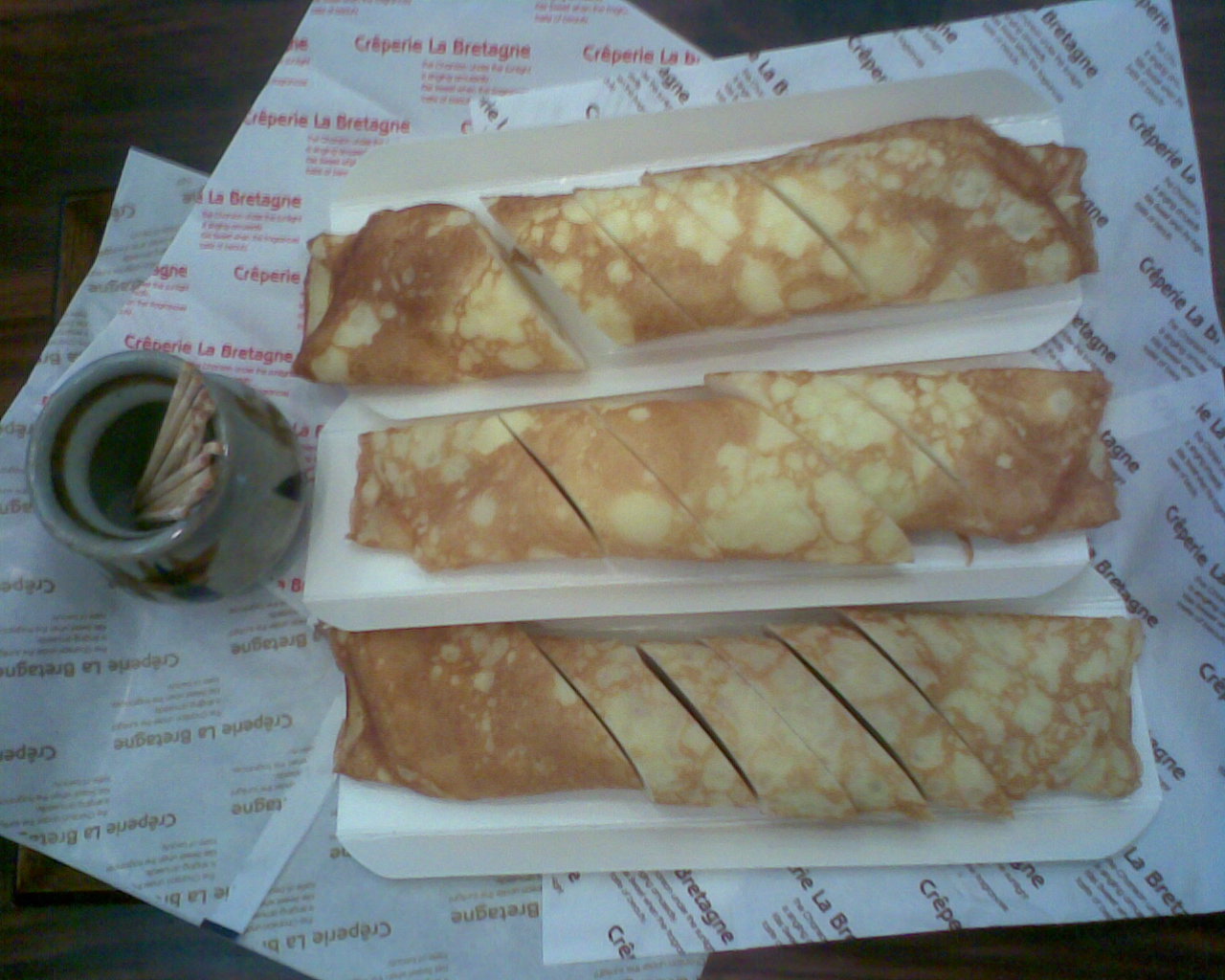This close-up image showcases three golden brown crepes, arranged horizontally in a top, middle, and bottom alignment. The crepes, which are sliced diagonally into thin strips, rest on individual white rectangular plates. The background features a white paper sheet imprinted with the phrase "CREPERÈ LA BRITAIN" and smaller text in French. Adjacent to the crepes on the left is a small green glass holder containing several toothpicks. The entire arrangement sits on a dark brown wooden surface, adding a rustic charm to the overall presentation.